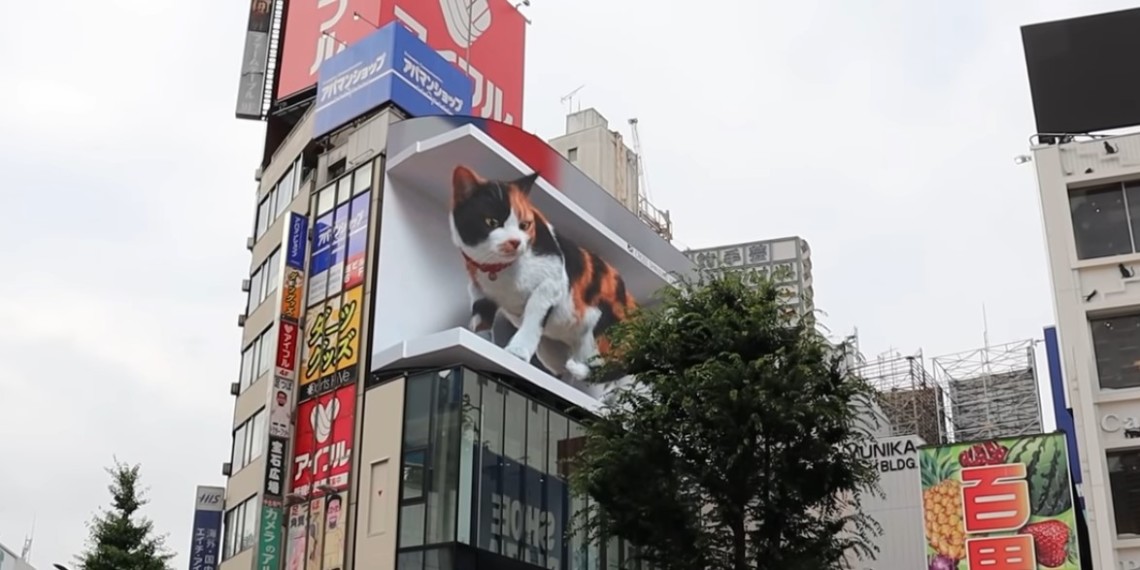This photograph captures a bustling scene in a Japanese city filled with towering buildings adorned with vibrant advertisements. Dominating the view is a technologically advanced 3D billboard that vividly displays a life-like calico cat. The cat appears to be moving on what looks like a white shelf, creating an impressive illusion of depth. It has a white underbelly and a striking fur pattern comprising black and orange patches, including a left orange ear and a right black ear. The cat also sports a red collar with a small bell. The building hosting this astonishing billboard is tan and features numerous windows. Flanking the main attraction are several colorful advertisements in hues of yellow, blue, red, white, and turquoise. Above the building, a large red billboard with white lettering stands out, while a fruit-themed advertisement with a green background and red lettering is visible towards the right. The sky overhead is gray and overcast, adding a muted backdrop to this vivid urban tableau, which also includes glimpses of trees in the foreground.